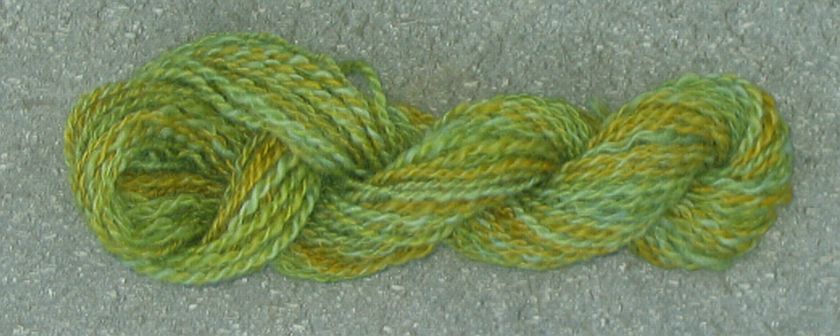This rectangular, horizontally oriented image features a predominantly gray concrete background that appears rough and scratchy to the touch. Spanning across the foreground of the photo, from left to right, is a thick, twisted yarn or rope. This rope is predominantly green, accented with streaks of yellow and orange. It fills most of the image, running horizontally and forming four prominent loops. 

In the center, the rope is tightly wound into a flowing knot, while the left side of the image shows the rope untangling and becoming loose, revealing individual strands. The right side remains tightly twisted, creating a stark contrast between the two ends. The setting suggests an outdoor environment, though the exact context or reason for the photograph remains unclear. Overall, the image showcases a striking interplay between the twisted, colorful rope and the stark, hard concrete background.